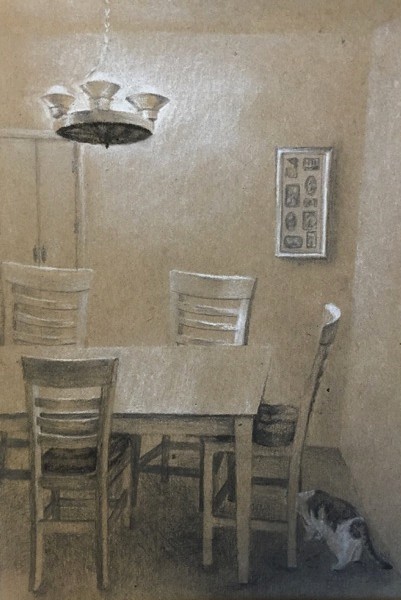This artwork appears to be a detailed charcoal or colored pencil drawing of a cozy dining room predominantly rendered in shades of beige and white with accents of black. The focal point of the image is a traditional blonde wood rectangular dining table, accompanied by four rung ladder back chairs, each with cushions. A black and white cat, its tail mostly black, is seen on the floor behind the chair at the head of the table. High above the table, a metal chandelier with upward-pointing lights dominates the ceiling, with three visible lights suggesting the presence of a fourth. The background showcases a minimalist yet charming atmosphere with tall, yellowish-beige walls adorned solely by a large rectangular frame, containing eight indiscernible photos arranged in four rows of two. There's also a discreet beige cupboard in the back left corner, merging into the wall, and possibly a door leading elsewhere. The illustration exudes a serene, muted ambiance, enhanced by the harmonious interplay of soft hues and thoughtful details.